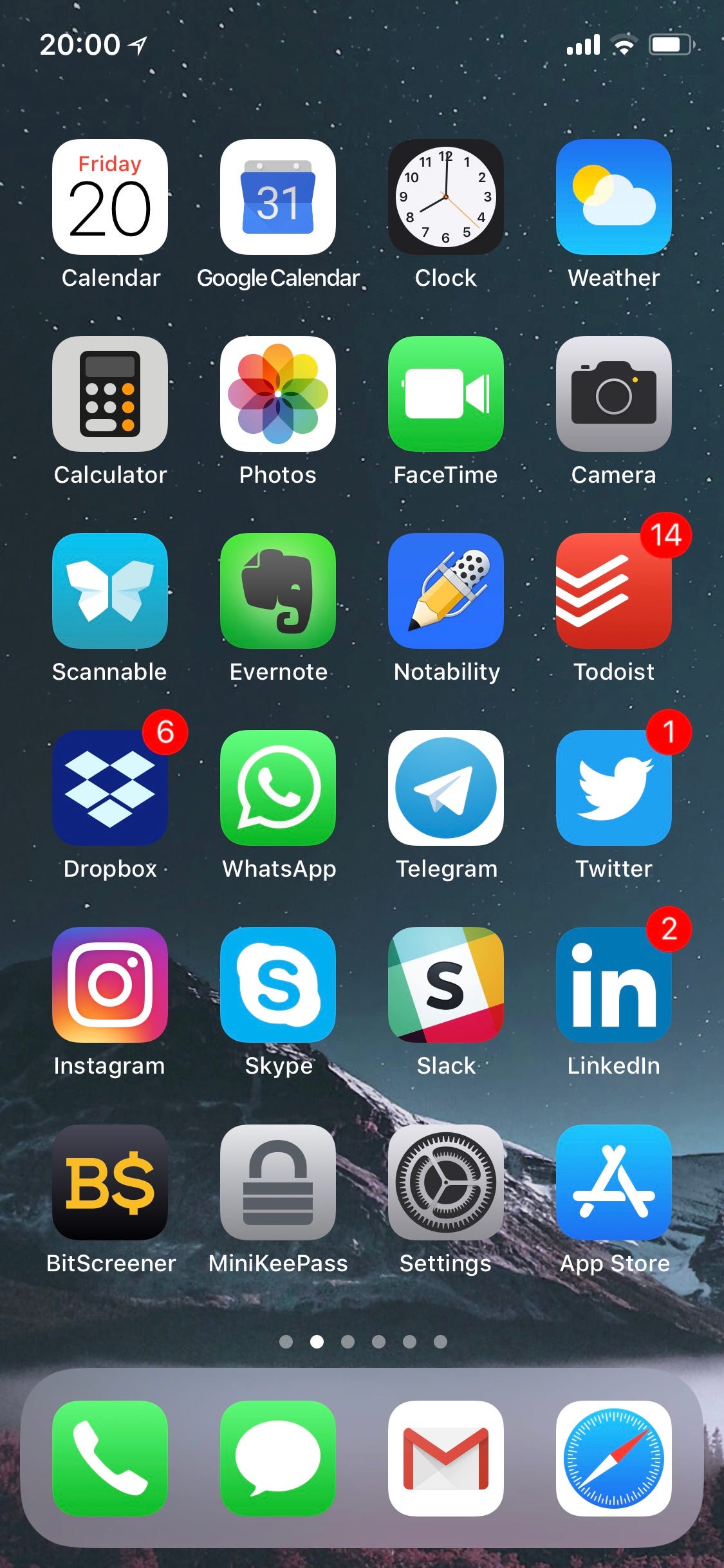The image is a vertically rectangular screenshot of a cell phone screen. At the top left, the time displays as 20:00, while the upper right corner shows the signal bar, WiFi, and battery icons. The screen showcases a grid of app icons, listed in vertical sequence from the upper left corner. The visible apps, from top to bottom, include Calendar, Google Calendar, Clock, Weather, Calculator, Photos, FaceTime, Camera, Scannable, Evernote, Notability, Todoist, Dropbox, WhatsApp, Telegram, Twitter, Instagram, Skype, Slack, LinkedIn, BitScreener, Mini KeePass, Settings, and App Store. Notably, four apps display notifications: Todoist with 14, Dropbox with 6, Twitter with 1, and LinkedIn with 2. At the bottom of the screen, four frequently used apps are docked: Phone, Text, Gmail, and Compass.